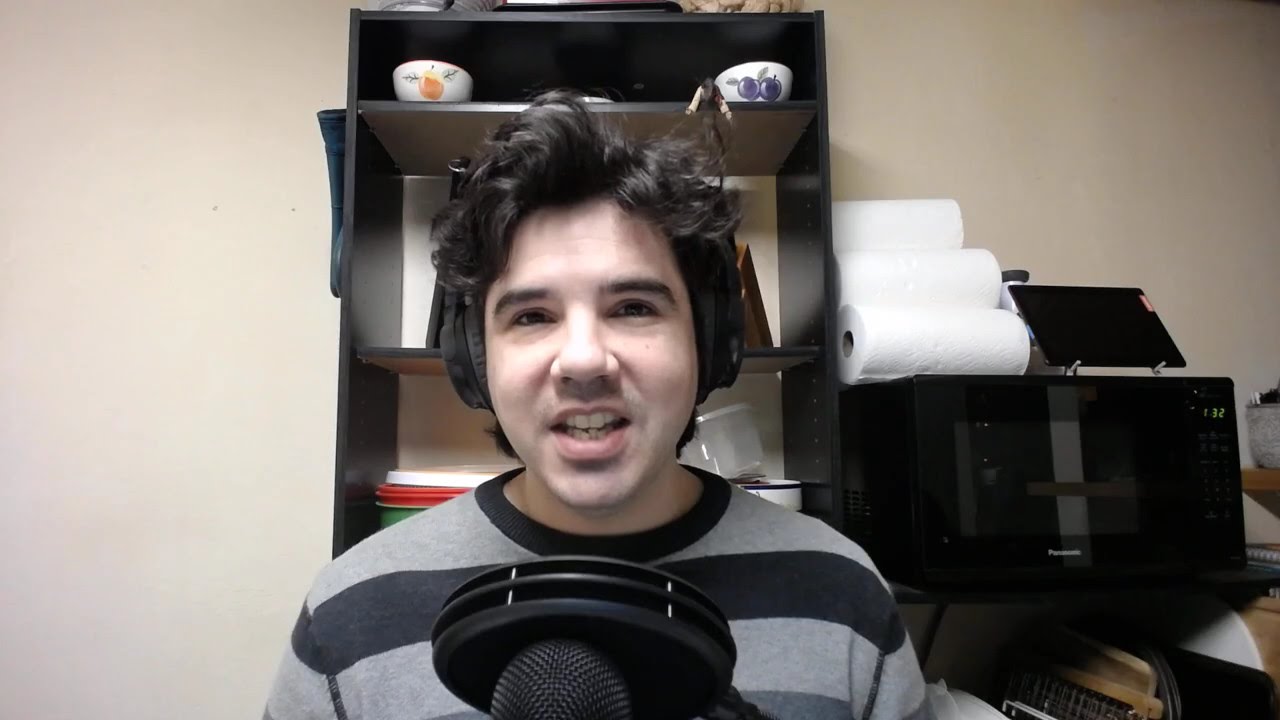A photograph captures a young man, likely in his late teens or early twenties, who appears to be speaking into a professional microphone with a circular disc in front of it. He has dark, fluffy hair and light skin, and he's wearing over-the-ear headphones along with a gray and black horizontally striped shirt. The man, whose mouth is open, revealing uneven bottom teeth, looks directly at the camera. 

Behind him, a beige wall provides the backdrop for a black cabinet with light brown shelves. On the topmost visible shelf, two white bowls flank the center—one holding an orange or peach on the left, and the other containing what appears to be purple fruit, possibly grapes or apples, on the right. To the right of the cabinet, a black printer or microwave is topped with a small monitor screen and a clock on its side, with rolls of paper or paper towels stacked atop it.